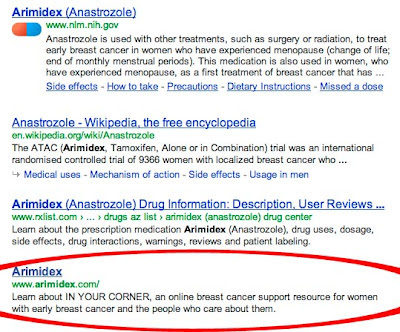The image is a screenshot of search results related to the medication Arimidex, also known as anastrozole. The first result, from the website nlm.nih.gov, explains that Arimidex is used alongside other treatments like surgery or radiation to treat early breast cancer in postmenopausal women. It further clarifies that menopause is the end of monthly menstrual periods. Additionally, the medication is described as a primary treatment for breast cancer in postmenopausal women, but the text is cut off beyond this point. The last search result, which has been circled, mentions "Learn about In Your Corner," an online breast cancer support resource for women with early breast cancer and their supporters.